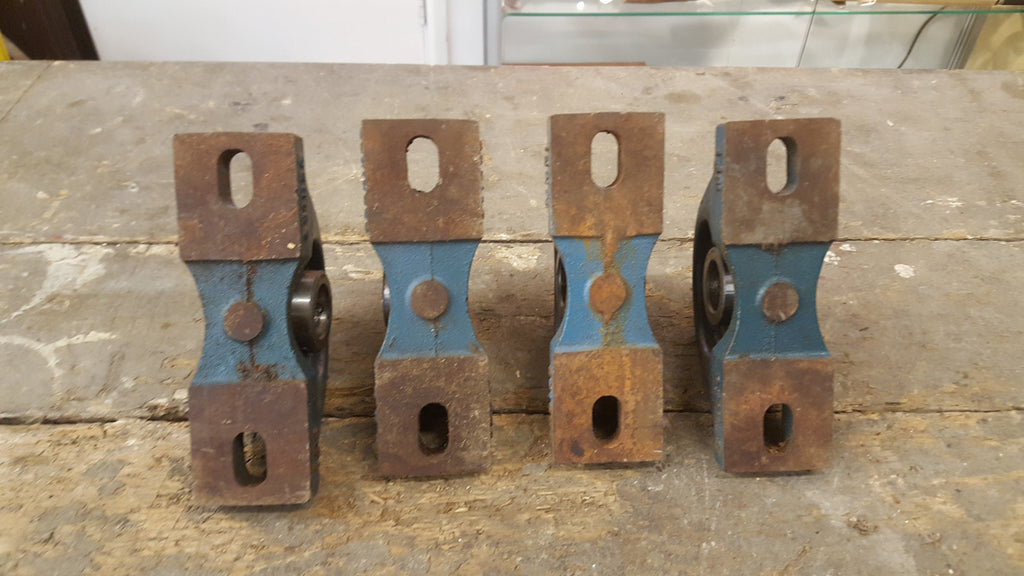The image depicts an old, weathered workbench, likely made of wood, characterized by its grayish-tannish surface, marred with scrapes revealing white patches and rust spots. Positioned on the table are four identical tools or implements, each composed of three main components. At the top and bottom are rusted, rectangular metal pieces featuring oval-shaped cutouts in a reddish-tannish hue. Sandwiched between these pieces is a blue wood-like section, distinguished by a round, protruding bolt of the same rusted bronze color as the rectangular parts. On either side of each implement is a silver, carbon steel circular attachment point, suggesting these items may connect to a machine or structure. In the far background, a white wall and part of a machine are visible, along with a wire descending on the right side. The overall impression is of a workspace dedicated to heavy or industrial use, with tools designed for securing pipes or serving as machine pedals.